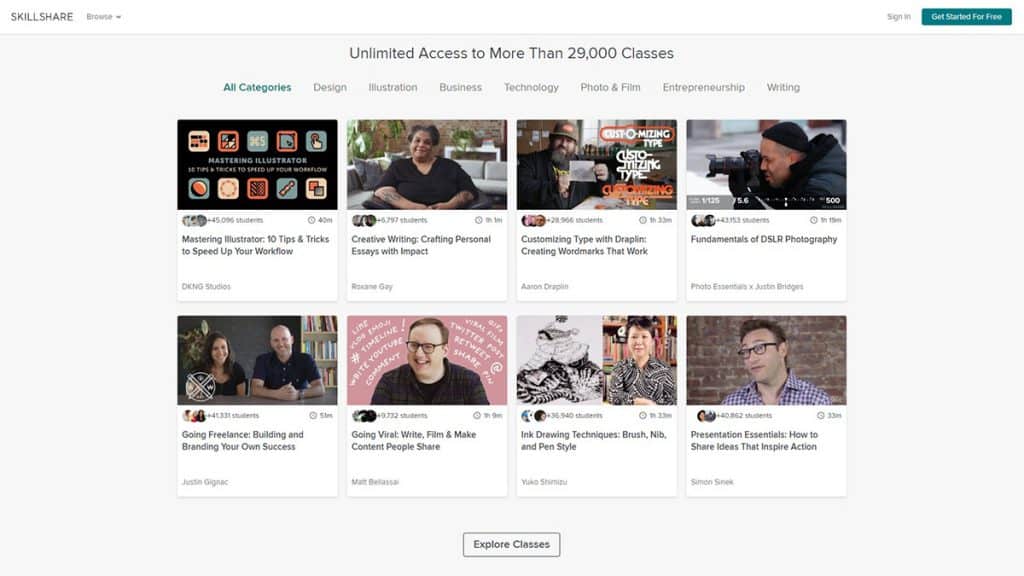A screenshot of the Skillshare homepage is set against a light background. In the top left corner, the Skillshare logo is displayed in black, capital letters. Next to it is the word "Browse" with a small black downward arrow. On the far right, in black, it says "Sign In" and next to it, a very dark blue rectangle reads "Get Started for Free" in white text.

The central portion of the page has a gray background with a prominent white message stating, "Unlimited access to more than 29,000 classes." Below this, in dark black text, it says "All categories." Seven categories are listed in gray text: Design, Illustration, Business, Technology, Photo & Film, Entrepreneurship, and Writing.

Underneath these categories, there are two rows of four photos each, presenting various class themes. The first photo is predominantly black. The second features a black woman looking directly at the viewer. The third photo shows a man with a large beard wearing a yellow-green hat, with some text on the image. The fourth illustrates a man dressed in black, facing left, and taking a photograph.

The second row starts with an image of a man and a woman sitting together and smiling subtly. The second image shows another man facing left, set against a pink background, dressed in black with words surrounding him. Next, there is an Asian woman seemingly sketching, and the final photo displays an Asian man standing in front of a brick background.